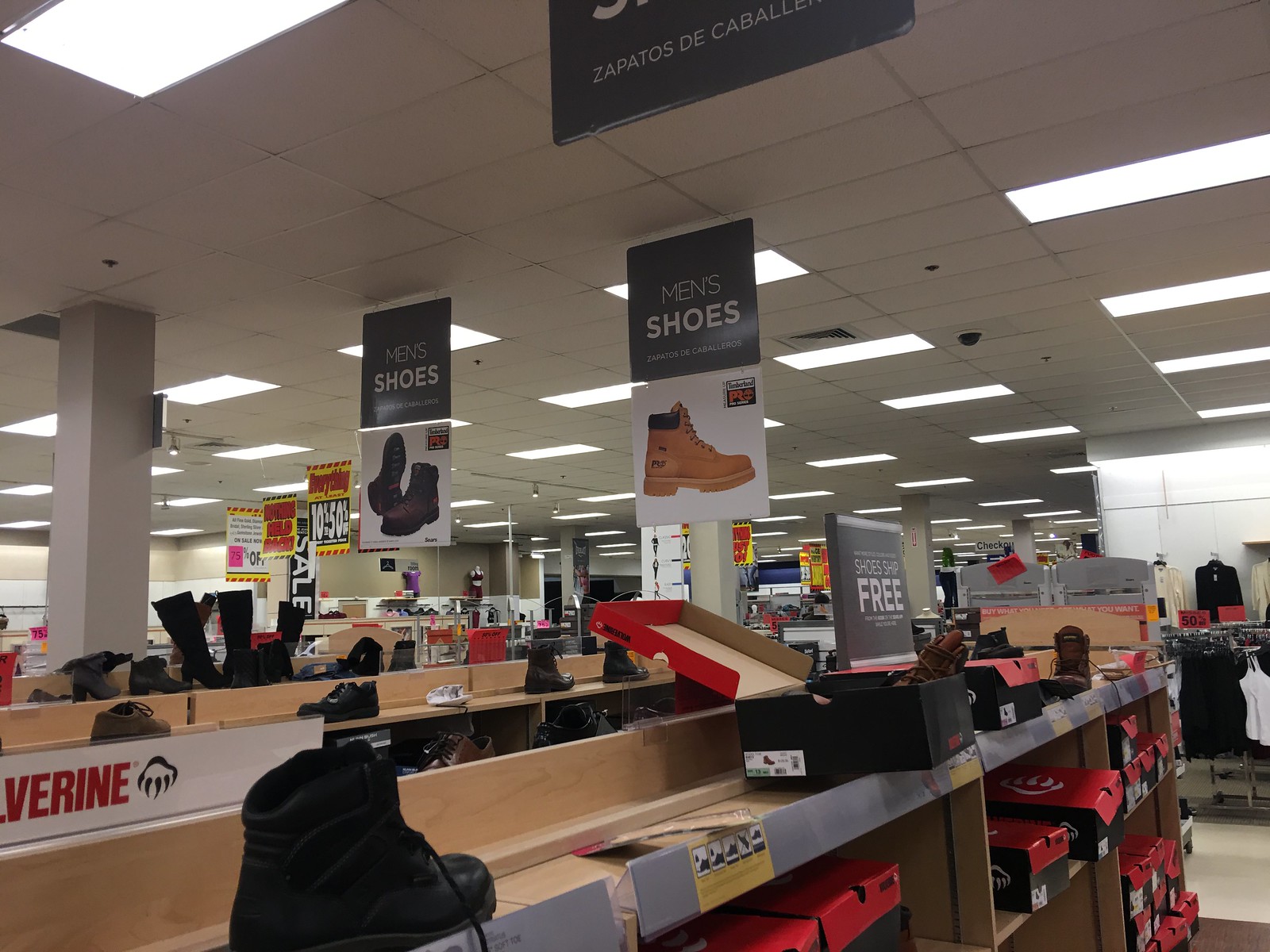The photograph depicts the interior of a department store, specifically in the men's shoe section. The picture captures an aisle flanked by shelves filled with various types of men's shoes and shoe boxes. The shelves are largely composed of light brown wood, with some described as gray along the edges. The shoe boxes visible are predominantly black on the bottom with red tops.

Hanging from the white ceiling, which features bright rectangular fluorescent lights and an air vent, are several signs indicating the presence of "Men's Shoes." One of the signs, partially visible, appears to read "Zapatos de Caballeros." These signs include images of different shoe styles, with black formal shoes on the left and brown hiking shoes on the right.

In the background, there are racks of clothing, with some jackets displayed on a white wall. Additional details in the image include a round shirt rack holding tank tops at the end of the aisle and a security camera mounted on the ceiling. The overall scene is brightly lit, indicating a well-illuminated retail environment.